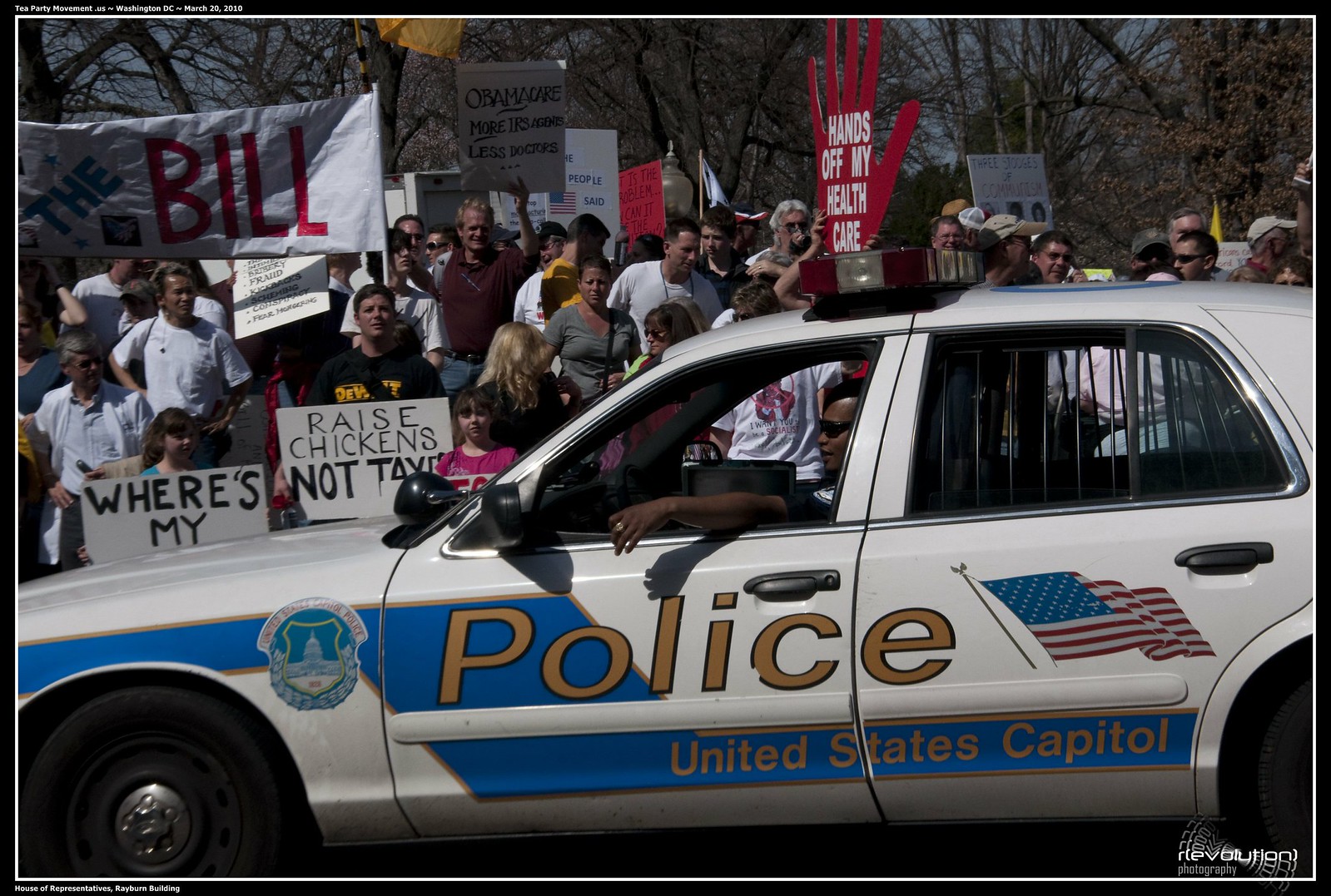The image captures a bustling protest in Washington, D.C., with hundreds of demonstrators of all ages, including children, gathered to voice their concerns. The crowd predominantly consists of African American individuals, many holding an array of signs reflecting their diverse messages and grievances. Notable signs include a large red hand declaring "Hands off my health care" and another saying "Raise chickens not taxes," pointing to taxation and healthcare as key issues. In the background, a sign reads "Obamacare is more IRS agents less doctors," indicating the protest likely dates back to the period between 2008 and 2016 when the Affordable Care Act, often referred to as Obamacare, was a hot topic.

A white police car from the United States Capitol Police, marked by a blue stripe and an American flag, is parked at the forefront of the scene, acting as a barrier to the protestors. The officer, an African American, appears relaxed yet vigilant, with his arm casually resting out the window, suggesting a warm day. The photo, taken from across the street, shows that the area has been cordoned off with barricades to prevent the crowd from spilling over into the road, maintaining order. Despite the density of the crowd, the atmosphere seems controlled and non-violent, with the officer simply observing the proceedings.